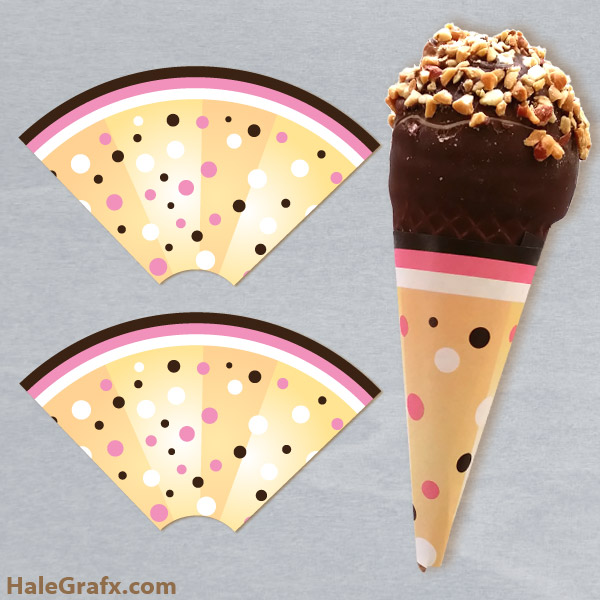The image showcases a product advertisement for ice cream cone wrappers from hailgraphics.com. The background is a solid gray. On the right side, there's a chocolate-dipped ice cream cone topped with nuts, wrapped in a decorative paper. This wrapper features a vibrant color scheme of alternating yellow and darker yellow, adorned with white, brown, and pink polka dots, and a border at the top in brown, pink, and white. To the left of the wrapped cone, two unfolded cone wrappers lie flat, revealing the same colorful pattern and border. At the bottom left corner of the image, "hailgraphics.com" is clearly printed in brown letters.